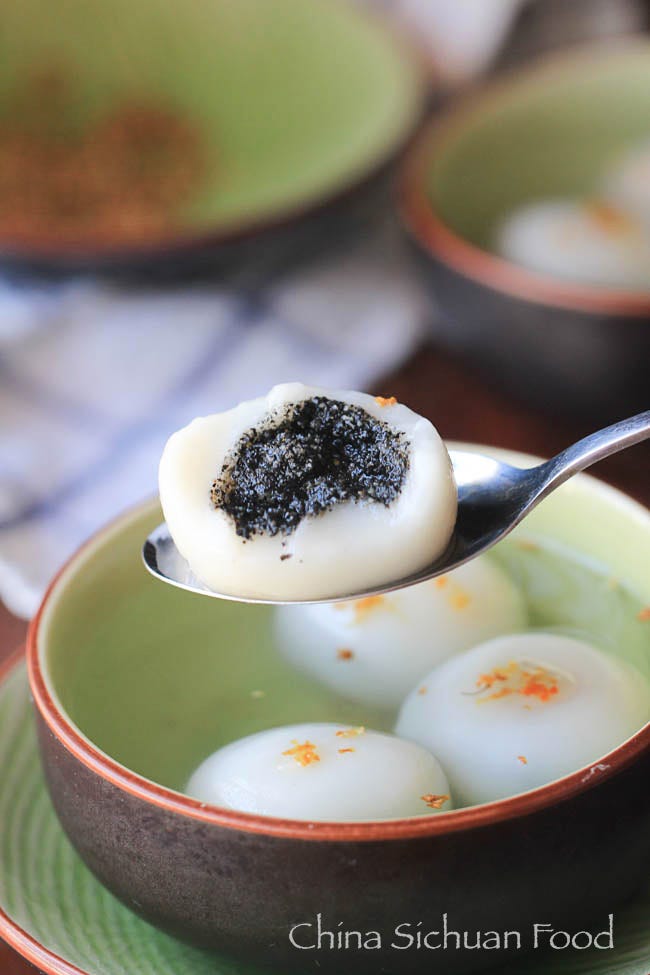The photograph showcases a detailed close-up of a bowl of traditional Chinese mochi-like dumplings, commonly associated with China Sichuan food, as indicated by the text at the bottom of the image. The central focus is a black bowl partially immersed in a larger green bowl, holding four white glutinous rice balls. One of the dumplings is cut open and held by a reflective silver spoon, revealing a black, slimy bean paste filling inside. The other three unopened dumplings are still submerged in a liquid within the black bowl. In the blurred background, there are additional bowls on a wooden tabletop, one identical to the featured bowl with similar contents, and another smaller bowl with indiscernible contents. The scene is grounded on a white and blue cloth, enhancing the rustic and authentic culinary presentation.